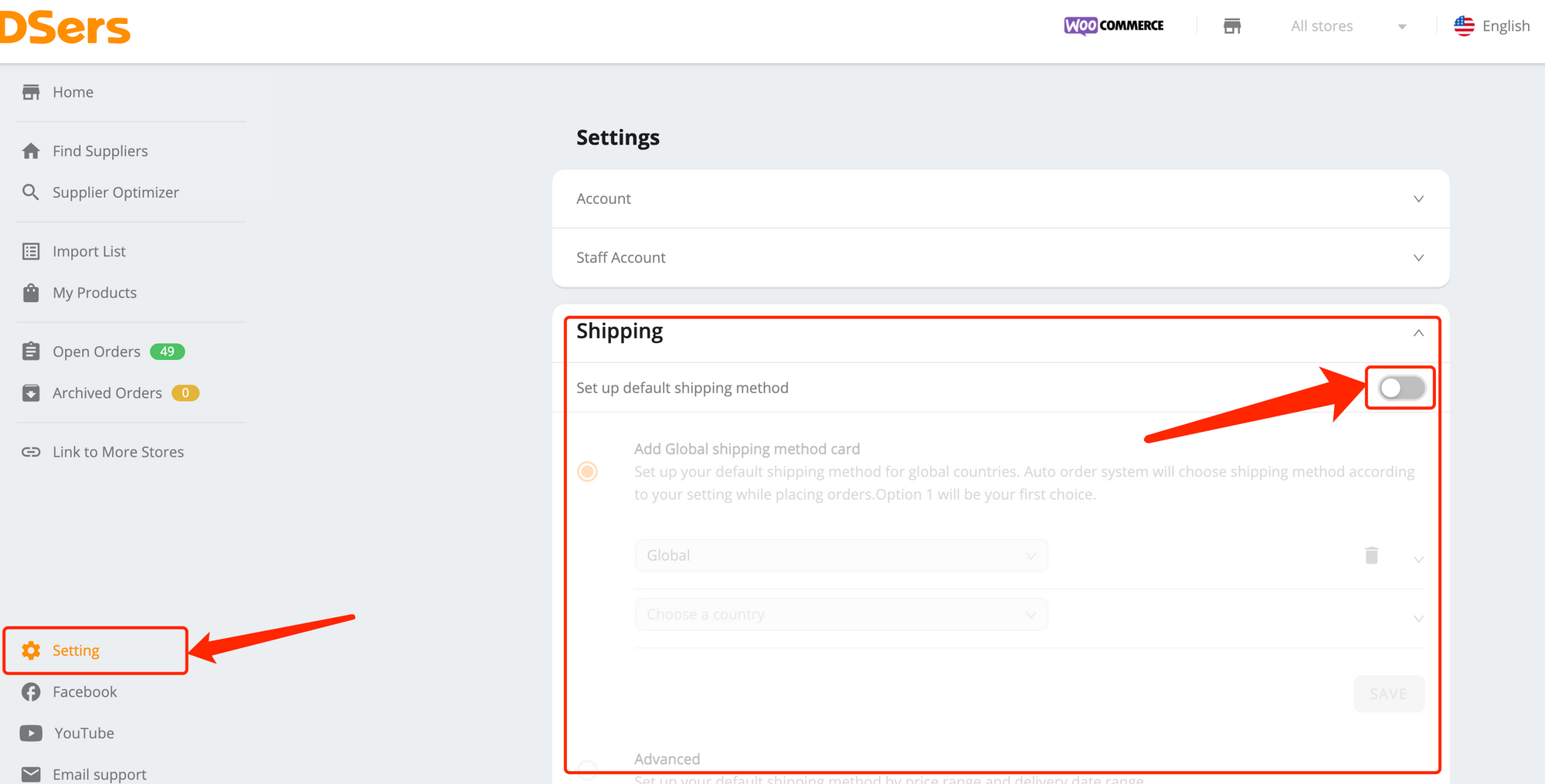This is a detailed caption for your image:

---

The web page features a dark gray top banner that reads "DSCR", indicating it as a platform where users can purchase web pages and domains. The header text is in orange, while the main page background is white. On the left-hand side, there is a vertical navigation menu.

The menu starts with:
1. **Storefront** (icon resembling a home)
2. **Find Suppliers** (icon of a magnifying glass)
3. **Supplier Optimizer** 
4. **Import List** (icon of a square with bulleted points)
5. **My Products** (icon of a shopping bag)
6. **Open Orders** (clipboard icon in black with white lines)
7. **Archived Orders** (square icon in black with a downward white arrow, accompanied by a circle with "0" in white)
8. **Linked to More Stores** (link icon)
9. **Settings** (gear icon)

Below the "Settings" option, there is an orange-bordered section highlighted by a red arrow, featuring icons for:
- Facebook (Facebook logo)
- YouTube (YouTube logo)
- Email support (generic envelope icon)

On the right-hand side, the page displays:
- **Settings** (bold black text)
- **Account** and **Staff Account** (two close rectangles with drop-down arrows)

The top right corner includes:
- A purple rectangle with the text "WOO" in black, followed by "Commerce" in bold black text
- A drop-down arrow labeled "All Stores"
- An American flag icon indicating the page is in English

A section below the "Settings" option, highlighted with a red rectangle, focuses on setting up shipping methods. It includes:
- "Shopping" in bold black text
- "Set up a default shipping method" with a slider, currently turned off, marked by a red rectangle and arrow
- Faded text within circles indicating "Add Global Shipping Method Card"
- An option labeled "Global" with a trash can icon
- Sections for "Change Inventory" and "Choose a country", both faded out
- A "Save" button in faded text
- "Advanced" section on the left-hand side

All visually highlighted elements incorporate clear graphical symbols, icons, and text to facilitate user navigation.

---